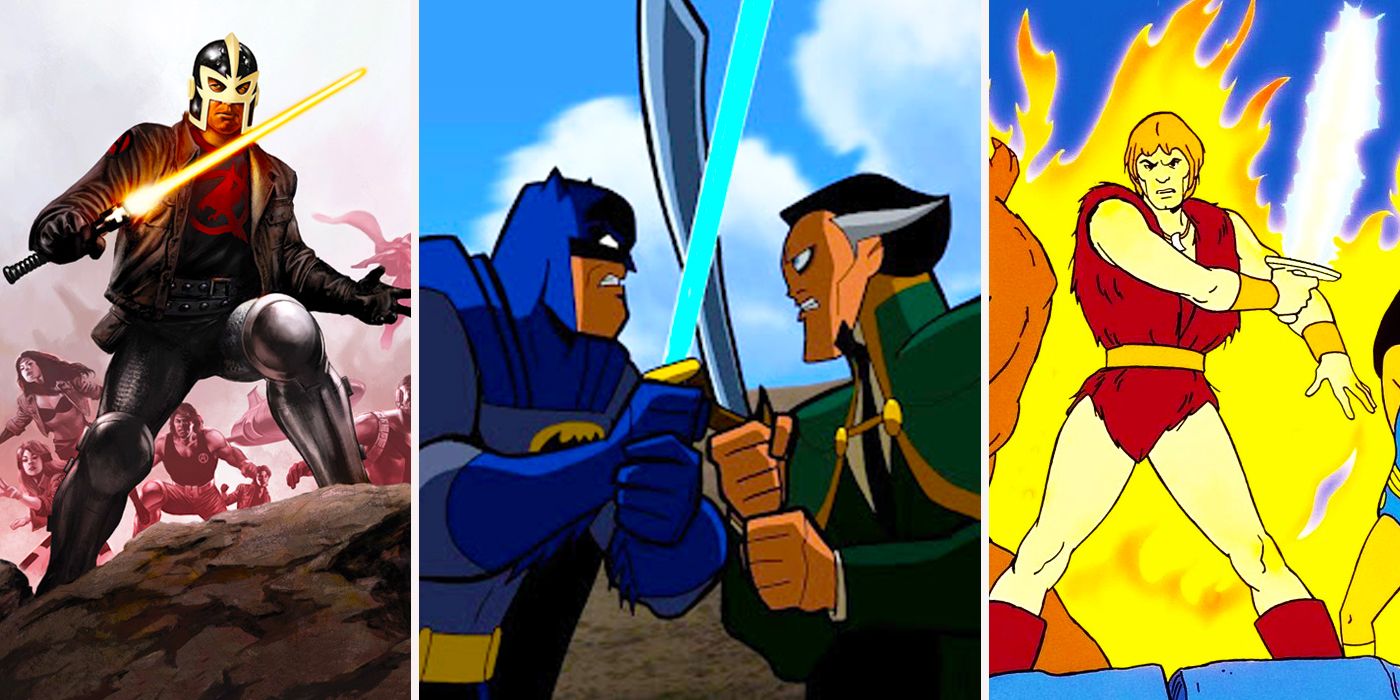This cartoon poster is divided into three detailed panels, each showcasing a unique character in action. 

On the left panel, the Black Knight from Marvel Comics stands heroically atop a rocky outcrop. Clad in a black leather jacket, tight black leggings with knee paddings, and a distinct headgear that is black with cream-colored areas around the eyes, he strikes a powerful pose. His left leg is bent at the knee, propped up on the rock, while his right leg remains straight. Holding a yellowish lightsaber in his right hand, his black shirt proudly displays a red letter 'A'. In the background, several other characters are rushing in the same direction, contributing to the sense of action and urgency.

The center panel features an intense standoff between Batman and Ra's al Ghul. Batman, in his iconic blue costume with black mask, belt, gloves, and boots, wields a shimmering blue laser sword. Opposing him, Ra’s al Ghul wears a green jacket and has a sword of his own. They are caught in a dramatic clash, their swords forming an 'X' between them. The backdrop is a vibrant blue sky filled with large white clouds, emphasizing the epic nature of their battle.

In the right panel, a muscular figure stands amidst a backdrop of roaring flames. He wears a striking red furry bodysuit with gold armbands and red boots, his bare thighs and legs adding to the bold appearance. Facing the viewer directly, he holds a saucer-like object emitting a brilliant white light. His intense stance and the dramatic flames behind him add to the figure's imposing presence.

Each panel captures dynamic moments, rich with detail and visual appeal, showcasing the unique elements and styles of the individual characters.